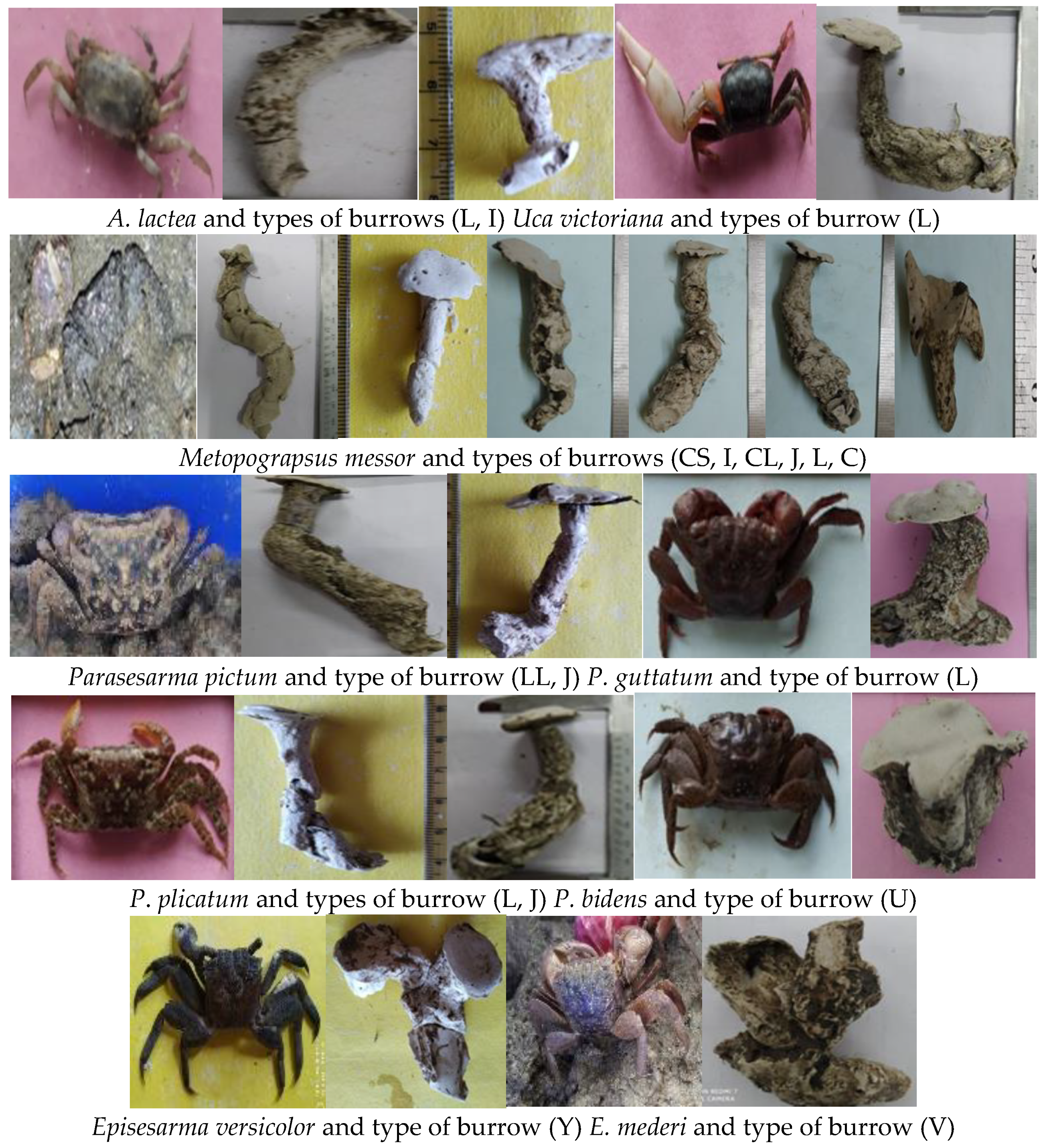The image features a series of color photographs arranged in five sections, each depicting various types of burrows and the crabs that inhabit them. The top row contains five photographs, followed by rows of seven, five, five, and four images. Each photo is accompanied by Latin text providing the scientific classification, such as "A. lactae," and detailed measurements of the burrows, indicating their length and width. The crabs vary in appearance, with some fully intact and others showing only their shells. The specimens are fossilized and come in diverse colors including gray, red, dark brown, chartreuse, pink, white, purple, and yellow. The layout and detailed captions suggest the images are from a scientific textbook. The focus is solely on the crabs and their burrows, with no other animals, people, structures, or vehicles present in the frame.